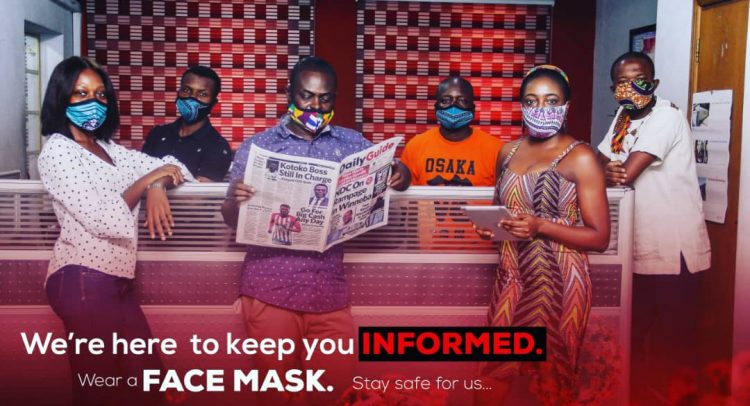**Detailed Caption:**

This image appears to be an advertisement, potentially a screenshot from a video on a computer or TV. The setting is defined by a distinct red background, enhanced by red lighting and a red overlay that sets an intense tone. In the foreground, six African American individuals—four men and two women—are standing around a dividing wall, creating a dynamic visual separation between them. All individuals are wearing face masks, emphasizing the ad's health safety message. 

On the left-hand side of the image, a woman with shoulder-length hair, a medium skin tone, and a blue face mask is wearing a white polka-dotted blouse paired with blue jeans. Adjacent to her stands a clean-shaven man in a blue shirt and slacks, intently reading a newspaper. 

The text, primarily in white at the bottom, proclaims, "We're here to keep you informed. Wear a face mask, stay safe for us..." The word "informed" is prominently highlighted in red within a black banner, and both "informed" and "face mask" are in bold, emphasizing the key messages. Notably, most of the individuals are looking directly at the viewer, creating an engaging and direct appeal. The specific style and elements of the advertisement suggest it may not originate from the United States, although this is a subjective impression.